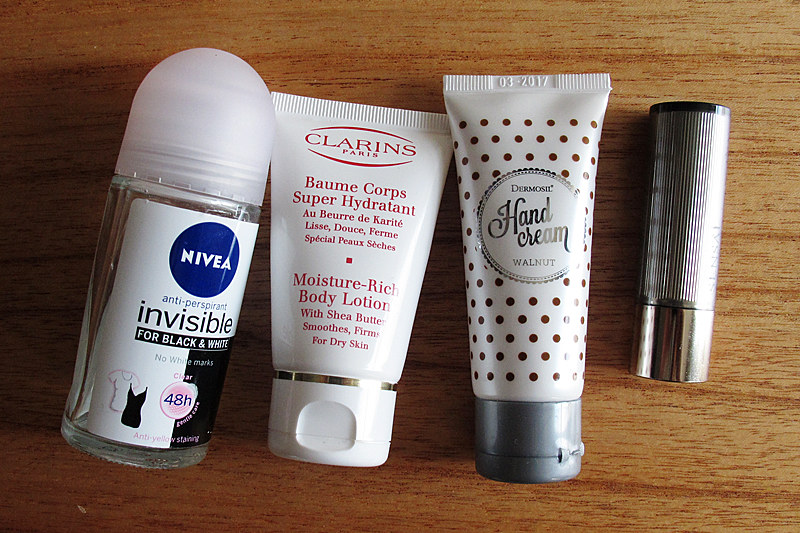In the image, four beauty items are meticulously arranged in a horizontal row on a wooden table. All items are placed lying down rather than standing upright. 

1. **Nivea Antiperspirant**: On the far left, there is a compact canister with an opaque white, rounded dome top. The canister features a white label adorned with a prominent blue circle, within which "Nivea" is written in white, uppercase letters. Below the circle, the text reads "Antiperspirant Invisible."

2. **Clarins Paris Moisture-Rich Body Lotion**: Positioned next to the antiperspirant, this item is housed in a white tube with its flip-top cap facing downward. The label states "Clarins Paris Moisture-Rich Body Lotion," providing a clean and sleek look.

3. **Dermasil Hand Cream Walnut**: The third item in line is another tube, similarly oriented with a cap-down position. It has a gray flip top, and the white body of the tube is decorated with gold polka dots. The label reads "Dermasil Hand Cream Walnut."

4. **Lipstick**: The final beauty item is a sophisticated lipstick. The lipstick is oriented with its applicator tip towards the top and the twisting mechanism at the bottom. The lower part of the tube features a metallic copper or silver hue with textured vertical stripes running around it, adding a touch of elegance.

Together, these items are neatly displayed on what appears to be a wooden table, providing a visually appealing arrangement of everyday beauty essentials.